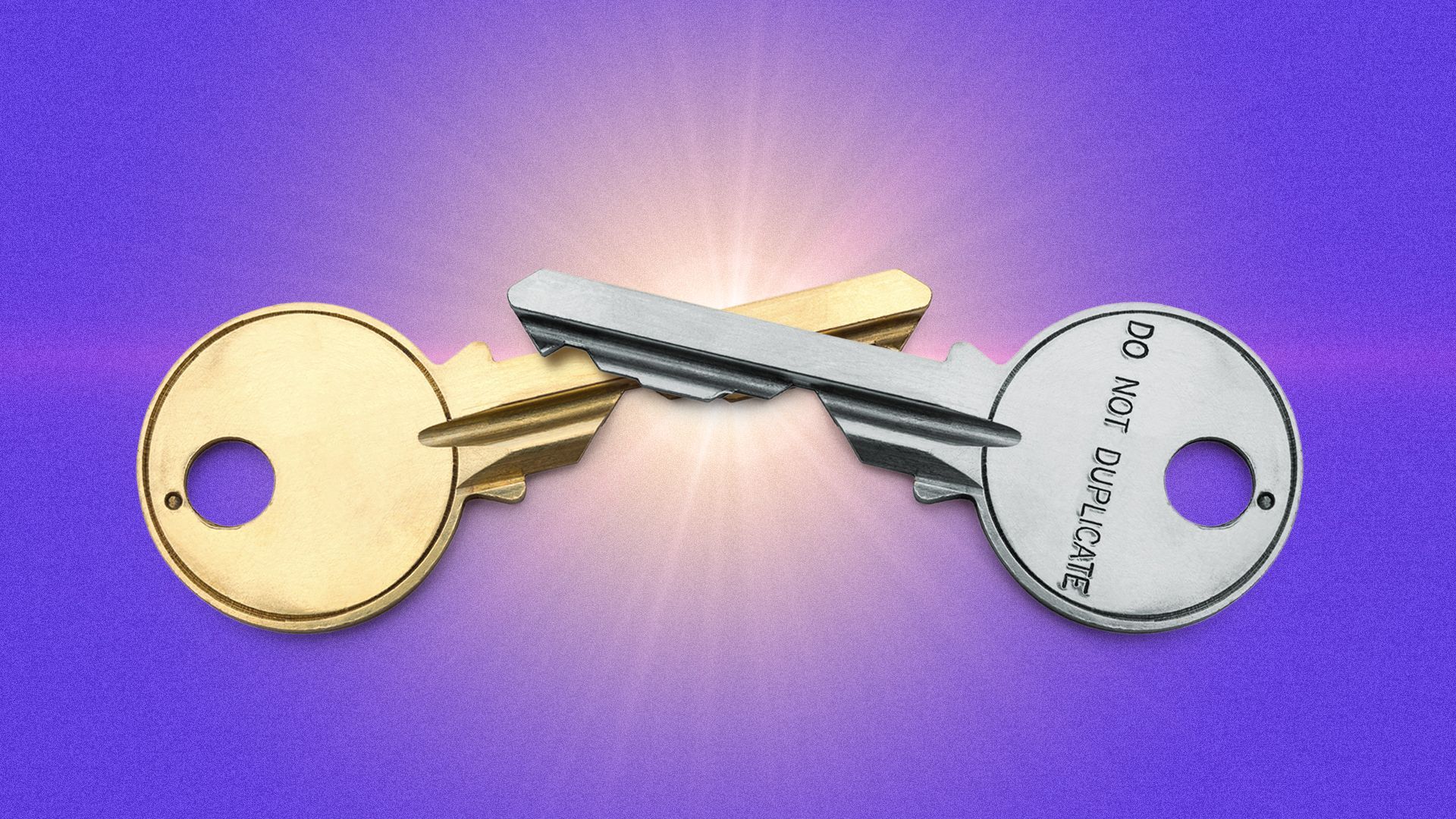The image depicts two overlapping keys forming a miniature X against a solid purple background, transitioning to pink where the keys intersect. The key on the right is silver, featuring the text "Do Not Duplicate" in black, with a circular head containing a large hole and a small circular indentation above it. This silver key has four teeth and is positioned with its head on the right side of the image. The overlapping key on the left is gold, mirroring the design of the silver key. Behind the keys, in the center, a radiant beam of light emits rays extending in various directions, blending yellow, pink, and orange hues. The scene is further enhanced by a subtle pink glow spreading horizontally in the background.